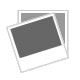This image captures a very old, unopened remote control for a ceiling fan and light, still encased in its original packaging. The remote, now yellowed from prolonged sun exposure, dates back to the early to mid-2000s. The AllFan branded device is ergonomically designed and beige-colored, featuring five buttons: four smaller oval buttons, likely for fan speed control, and a larger button for the light function. The packaging is a beige plastic shell, often requiring scissors to open, and includes a black and yellow poster displaying a ceiling fan and light. The text on the packaging specifies that the remote is suitable for all brands of ceiling fans with a detailed list of features. Despite its age and discoloration, it's assumed to still function, though it's outdated by modern standards. The remote's ergonomic design suggests it would sit comfortably in the hand.